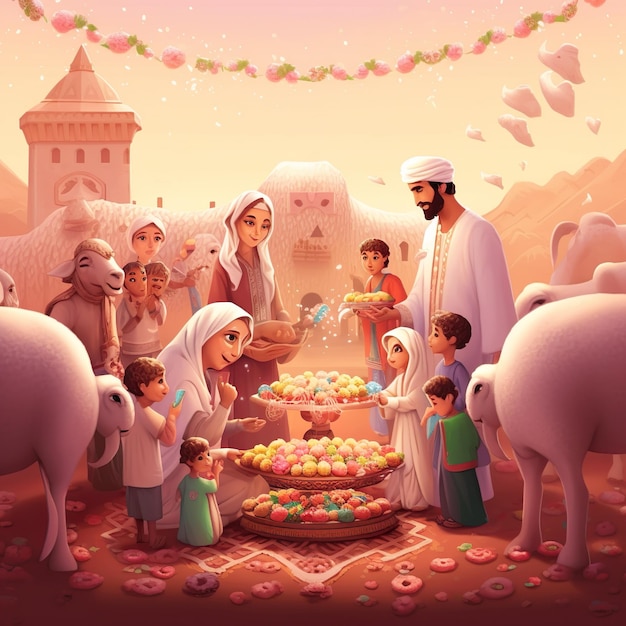This digital illustration, set in a Middle Eastern backdrop with buildings faintly visible in the background, captures a celebratory scene of a family gathered around a festive array of treats. Central to the illustration is a three-tiered dessert holder, adorned with colorful round balls in shades of yellow, pink, green, brown, and blue. Women, children, and one man are attentively gathered around, with a person in the background approaching with another basket of treats. The scene is enriched with the presence of white sheep surrounding the group, and scattered donuts on the ground add to the festive atmosphere. Above them, a garland of pink flowers and green leaves hangs, contributing to the celebratory ambiance. The overall palette of the image features pale browns and other soft hues, adding a warm and inviting feel to the illustration.